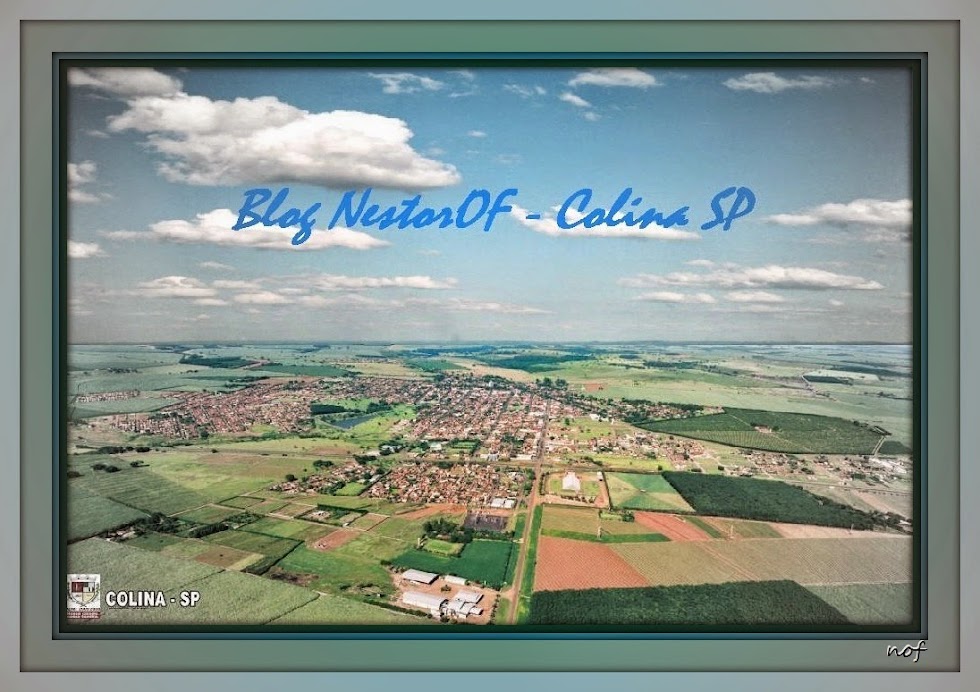This image features a large aerial photograph, occupying the entire frame, capturing a detailed and expansive view from above. The photo encompasses a diverse landscape of agricultural fields in varying shades of green and brown, intermixed with residential homes and developed areas. The top of the image showcases a clear blue sky dotted with fluffy white clouds. The composition draws the eye centrally, highlighting the spread of farmland and housing developments below.

The text "Blog Nestor OF Colina SP" is prominently displayed in a blue, cursive font near the top of the image, lending an elegant touch, while the bottom left corner features "Colina SP" in white alongside a logo. The overall palette merges calming blues and bright whites of the sky with the earthy greens and browns of the land, enhanced by touches of orange. The entire scene is encapsulated within a photo frame, presenting the image as a scenic and detailed snapshot, possibly a painting-like photograph, offering a serene overview of the landscape below.